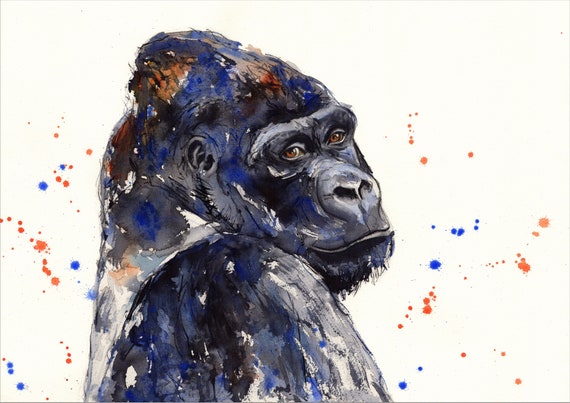The image is a highly detailed painting of a gorilla with a captivating artistic style that merges elements of digital and watercolor painting. The gorilla, depicted in shades of black and gray, dominates the center of the piece, occupying approximately 80% of the canvas, and is positioned at an angle with its head turned slightly to look toward the viewer. This playful expression gives the impression that the gorilla is deep in thought or observing something with a pleasant demeanor. The background of the image is white, yet it is intricately adorned with splashes and specks of blue and orange paint that scatter across both the background and the gorilla itself, creating a dynamic and visually engaging composition. These splashes also blend subtly into each other, enhancing the watercolor effect. There is no text within the image, allowing the viewer to fully appreciate the complexities and nuances of the painting.